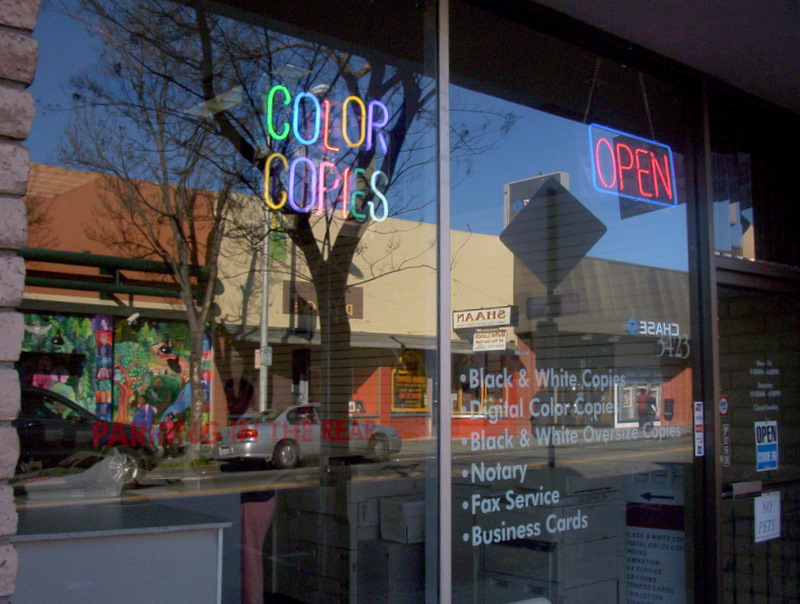The image depicts the entrance of a small, family-owned print shop, characterized by its predominantly glass façade that extends from ceiling to floor, allowing reflections of neighboring establishments such as a Chase Bank, a Muslim restaurant, and a toy store. On the left side, the shop features two large glass windows. The leftmost window displays a vibrant LED sign in two lines—spelling "COLOR COPIES," with each letter in different hues: the first line uses green, light blue, red, yellow, and purple; the second line employs yellow, purple, pink, red, green, and white. The right window includes an "OPEN" sign hanging from the ceiling inside the shop. Below these windows, a series of booths inside the store offers various services: black and white copies, digital color copies, oversized black and white copies, lottery tickets, fax services, and business cards. The entrance door, set in a black metal frame with a push bar, also bears an "OPEN" sign, highlighting the store's operational status.